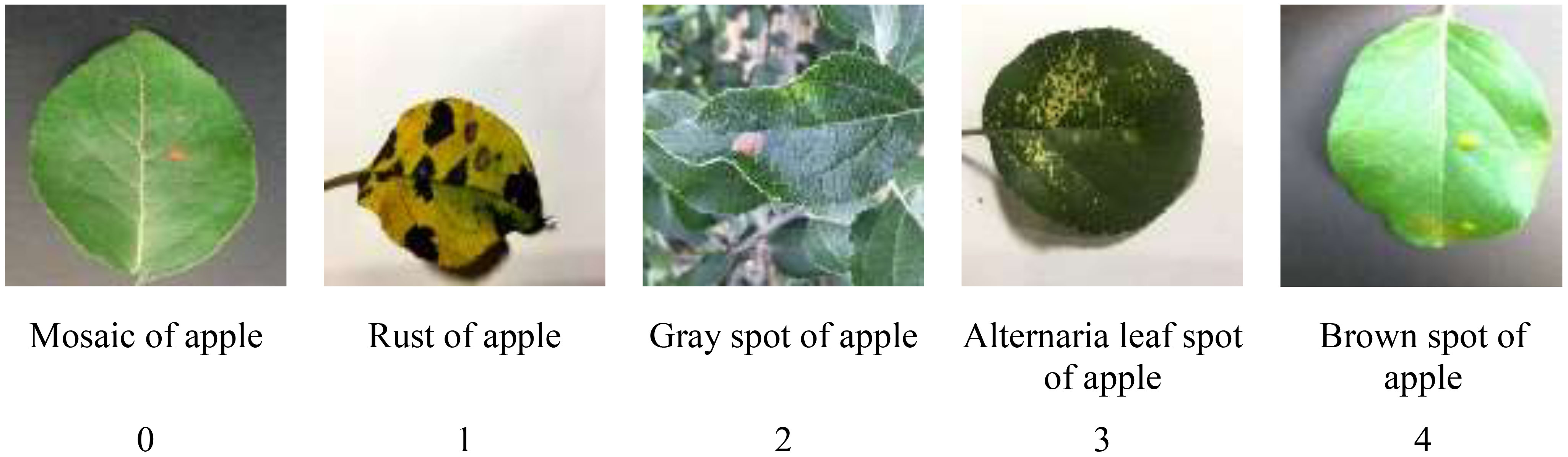The image is a scientific, rectangular composition featuring five horizontally aligned squares. Each square contains a detailed image of an apple leaf, displaying various diseases. The squares are numbered sequentially from 0 to 4 and each is labeled with a specific type of apple leaf disease. 

Starting from the left, the first square (0) is labeled "Mosaic of Apple" and shows a bright green leaf with a small pink dot. The second square (1) is labeled "Rust of Apple" and features a yellow leaf heavily speckled with very dark, almost black spots, and has frayed edges. The third square (2) is labeled "Gray Spot of Apple" and depicts a pointed green leaf with a pink spot, amidst some other leaves. The fourth square (3) is labeled "Alternaria Leaf Spot of Apple" showing a dark green, round leaf with lighter colored splotches. The last square (4) is labeled "Brown Spot of Apple" and displays a bright green leaf with some yellow spots. Each leaf varies in color, texture, and the nature of the spots or discolorations, effectively representing different stages and types of apple leaf diseases.